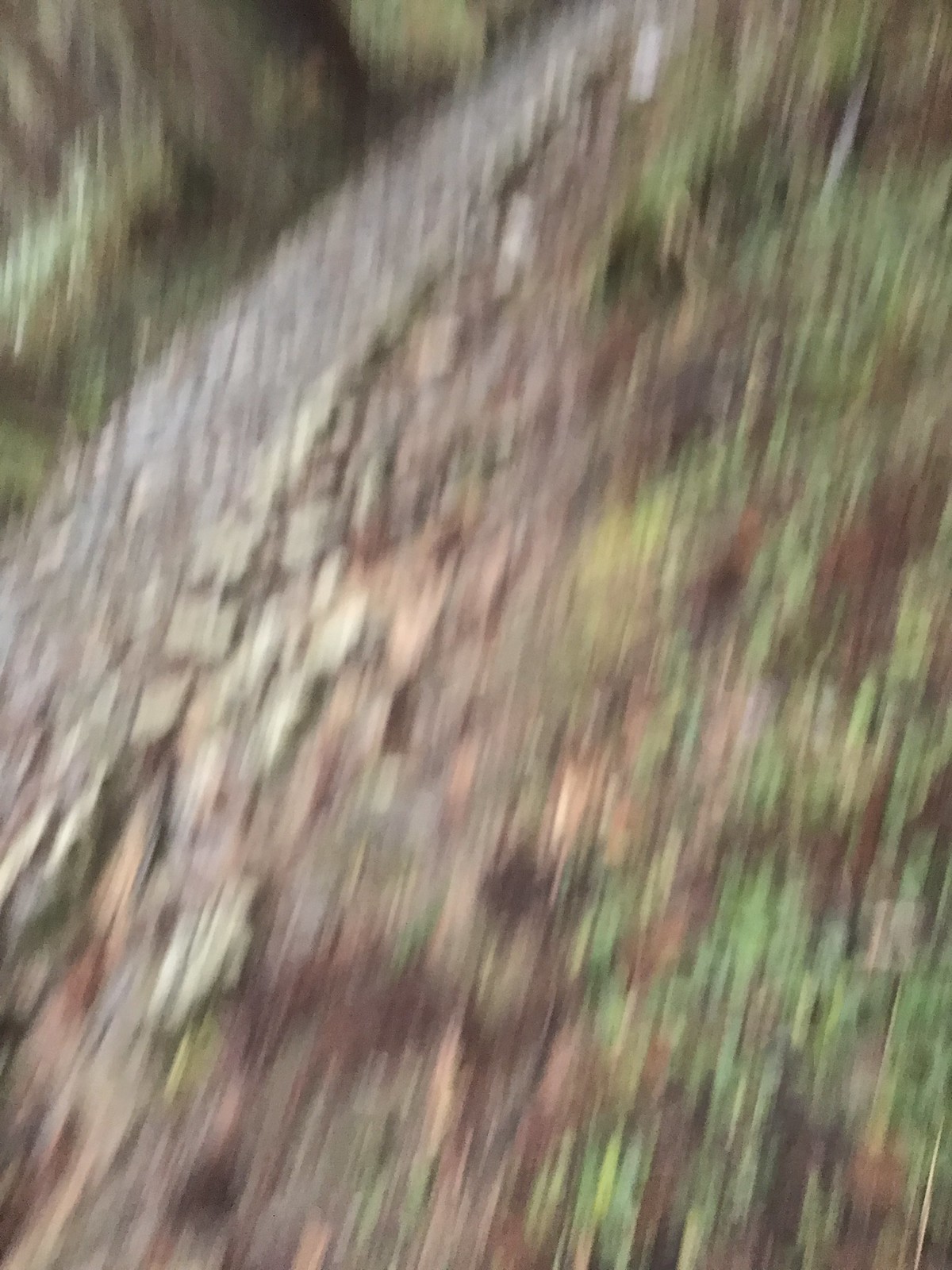The image depicts a blurry and out-of-focus shot of a forest floor. The scene features a wooded terrain with a discernible pathway starting from the bottom left and winding its way to the top right. Greenery is visible in patches towards the top left and along the right side, suggesting the presence of modified plants with green leaves. The right section of the image also contains stones amidst the dirt, which leads up to more green vegetation. The photograph appears to be an action shot, capturing a dynamic movement from top to bottom, adding a sense of motion to the otherwise still forest landscape.